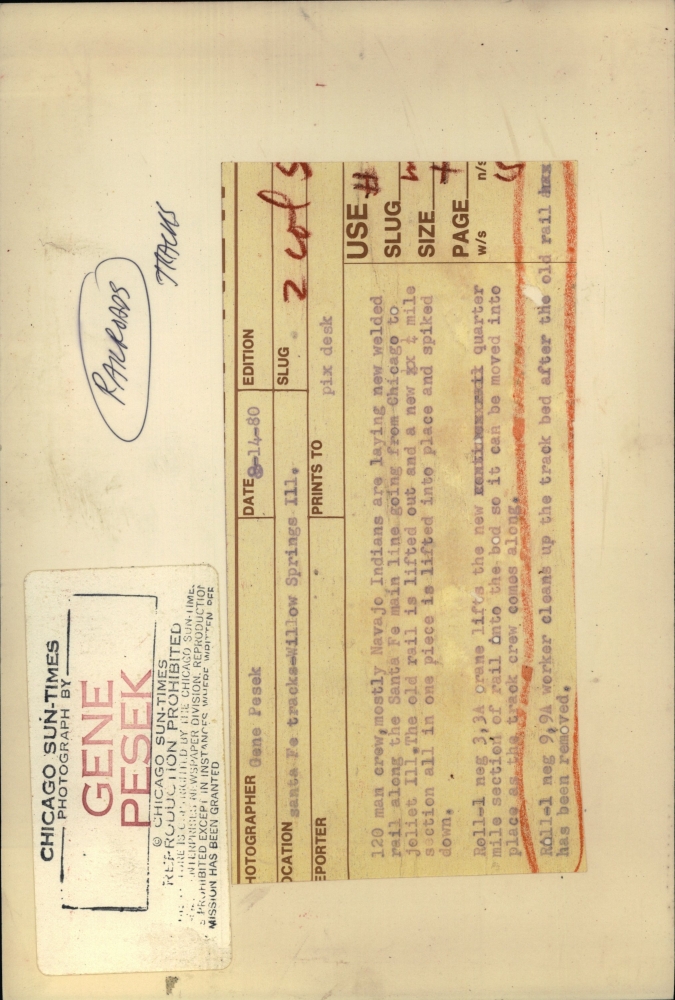This detailed image depicts the reverse side of a photograph taken on August 14, 1980, for the Chicago Sun-Times by photographer Gene Pesek. The document, aged to a yellow hue and framed in off-white, has been rotated 90 degrees counterclockwise, making it slightly difficult to read. It prominently features a stamped sticker that reads "Chicago Sun-Times photographed by Gene Pesek" in red all caps within a black outlined rectangle, along with "copyright Chicago Sun-Times reproduction prohibited" below it. The document provides extensive details including the photographer's name, the date, and location—Santa Fe Railroad in Willow Springs, Illinois. It mentions that the photo captures a 120-man crew, mostly comprised of Navajo Indians, laying new welded rail along the Santa Fe mainline from Chicago to Joliet, Illinois. The description highlights the labor-intensive process of replacing old rail with new rail sections, lifted into place in one quarter-mile lengths and then spiked down. Other fields, such as the reporter's name and additional technical details, remain blank or hard to decipher due to the document's age and coloring. Overall, the document is an informative artifact, providing insight into the meticulous documentation practices for newspaper photography in 1980.